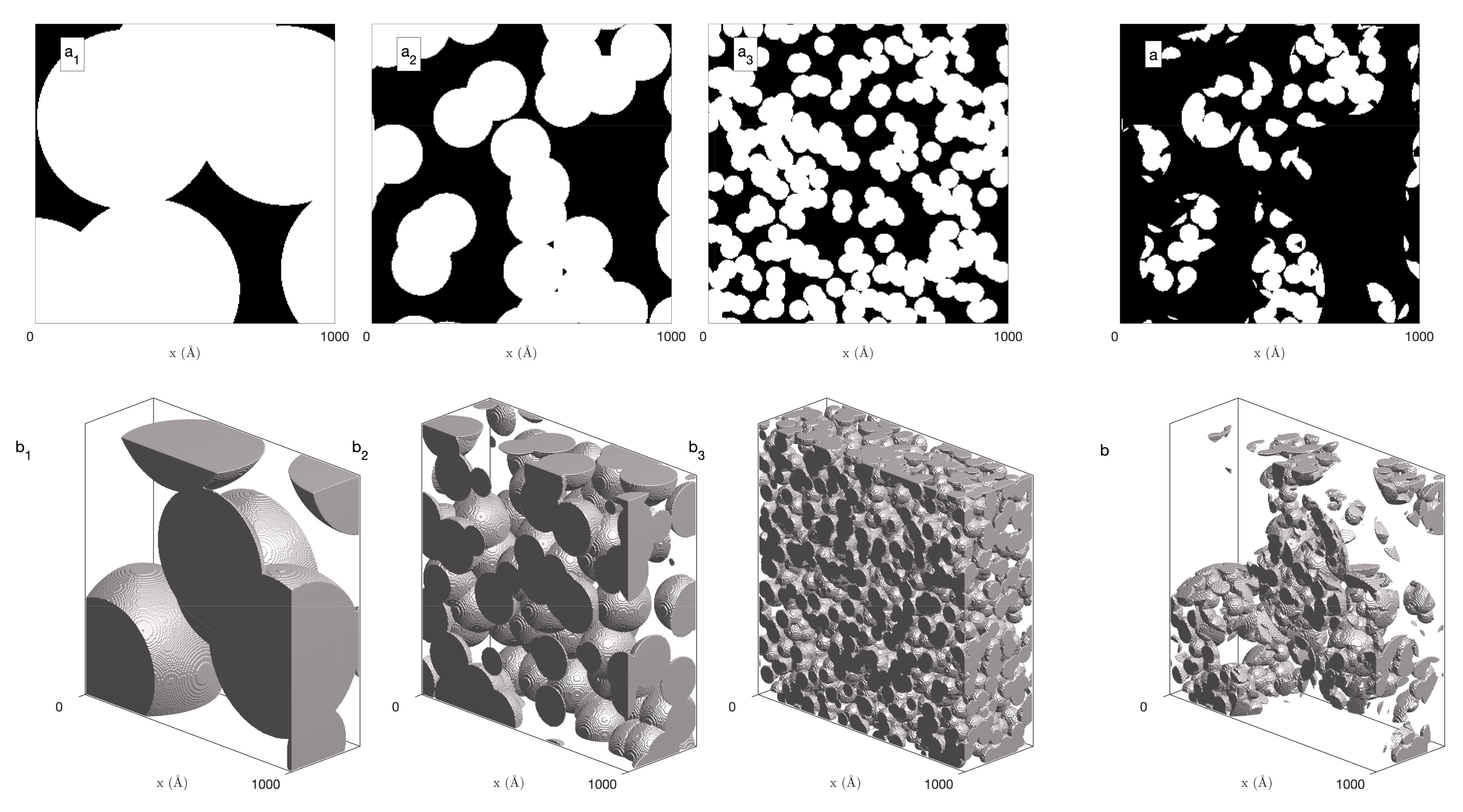The image features a scientific and biological theme presented through a grid of eight individual panels, split into two rows. The upper row showcases four black-and-white, two-dimensional images, each displaying various arrangements of white shapes against black backgrounds. The first panel on the upper left contains large white circles, some extending beyond panel borders. Moving rightward, the panels display progressively smaller white circles, intensifying the black backdrop. The final panel on the upper right features irregular white shapes, deviating from the consistent circular forms of the others. 

The lower row mirrors the upper images, transforming them into three-dimensional representations with gray objects against white backgrounds. Each 3D image corresponds directly to the 2D view above it, depicting similar formations of semi-circles and spheres. These shapes appear compressed within an invisible 3D frame, creating an angled effect. The lower images retain the structural essence of the upper panels, enhancing depth and spatial understanding between the top 2D and bottom 3D illustrations. Labels surround each panel, providing context for these scientific visualizations.